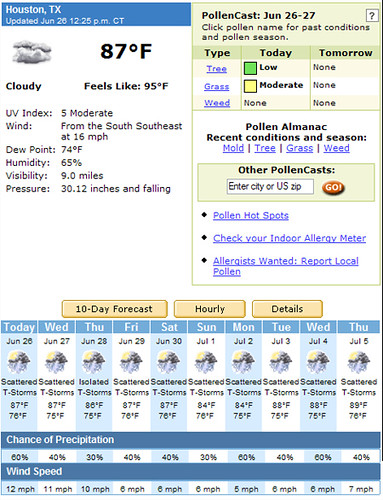**Screenshot of a Weather Webpage for Houston, Texas**

The webpage provides a current weather snapshot and forecast details for Houston, Texas. In the upper left-hand corner, a blue bar with white text indicates the location "Houston, Texas" and the last update timestamp, "June 26, 12:25 PM CT."

**Current Weather Overview:**
- **Icon:** A small graphic depicting clouds.
- **Temperature:** 87°F
- **Description:** Cloudy
- **Feels Like Temperature:** 95°F
- **Additional Weather Conditions:** Various details outlined below the main temperature box.

**Pollen Information:**
- **Heading:** Pollen Cache (June 26-27)
- A prompt encourages users to click on pollen names for past conditions and pollen season information.
- **Table Columns:** Type, Today, Tomorrow
  - **Types of Pollen:** Tree, Grass, Weed
- Below the table, additional sections provide details of the pollen almanac and recent conditions and seasons for mold, tree, grass, and weed.
- **Search Function:** Allows users to look up the pollen cache based on city or US ZIP code.

**Forecast Section:**
- At the bottom of the page, users can access the forecast through buttons labeled "10-day forecast," "Hourly," and "Details" (orange buttons with black text).
- The 10-day forecast starts from June 26 and extends to Thursday, July 5.
  - **Daily Forecast Details:** Includes an icon representing the weather type, the high and low temperatures, the description of the weather, the chance of precipitation, and wind speed for each of the 10 days.

This detailed caption provides comprehensive information about the weather and pollen conditions in Houston, Texas, as displayed on the captured web page.